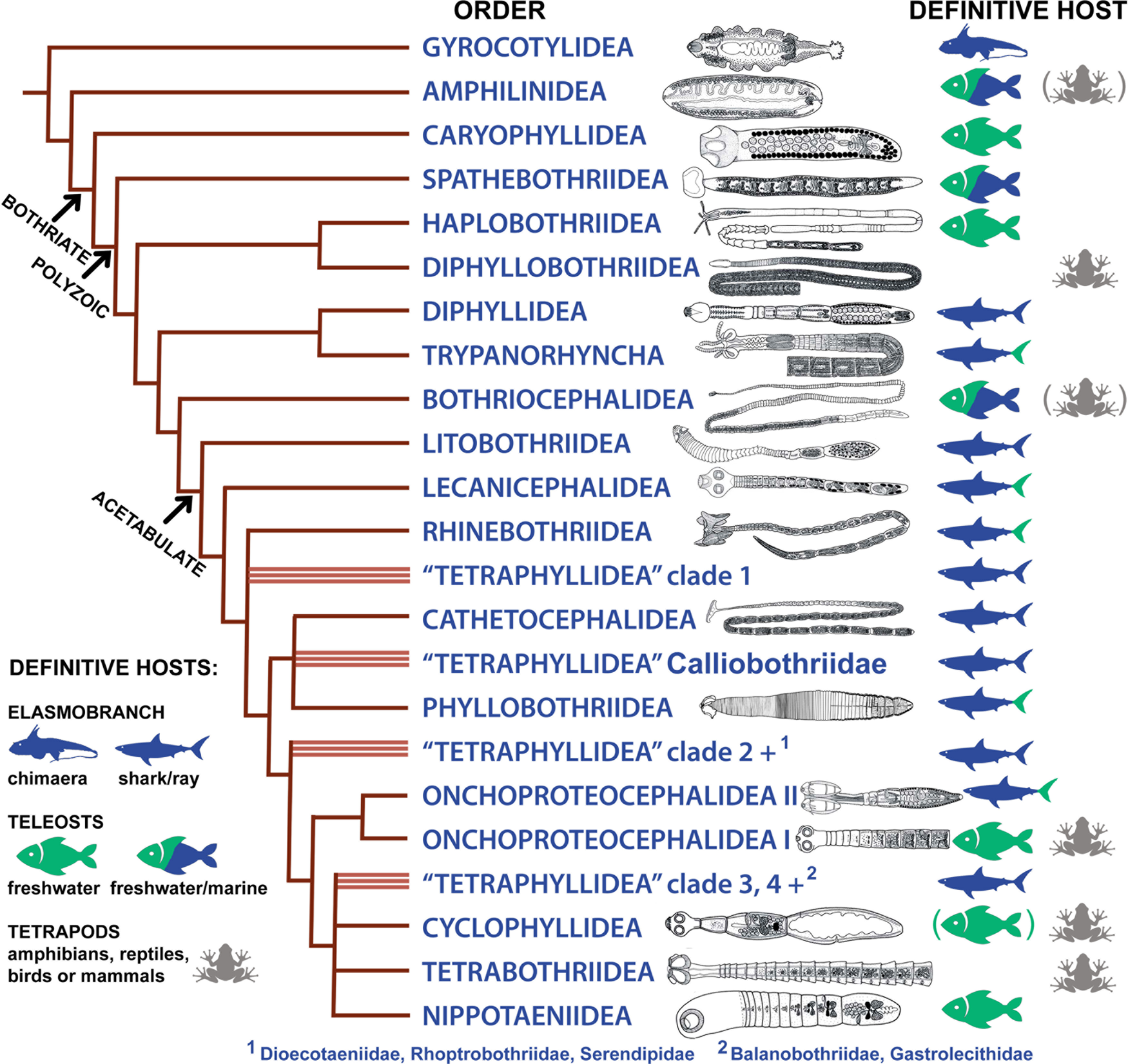The detailed chart starts from the left-hand side with the title "Definitive Hosts" written in blue letters along the top. There are red lines emanating downward, pointing to the various orders listed in blue. The chart features approximately 20-21 names in all capital blue letters, each indicating different types of fish, sea creatures, and other animals. This section spans from the top of the chart to the bottom.

In the middle column, there are various gray images of these sea creatures, featuring line drawings that depict different species, such as sharks and other marine animals. The column is organized with definitive hosts for each species, listed from top to bottom. The grid is divided with a mix of blue and green images indicating whether the creatures are freshwater, marine, or a combination of both.

To the far right of the chart, there are additional images of sea creatures positioned in two groups of three: one group at the top and another at the bottom with some spacing in between. Below this section, blue letters provide descriptions of the images from left to right.

Additionally, the chart includes the term "E-L-A-S-M-O Branch" and "C-H-I-M-A-E-R-A," picturing these categories along with sharks and rays. It mentions that T-E-L-E-O-S-T-S, denoted in green, signifies a freshwater fish, with another fish marked as partly blue and green for freshwater/marine environments. In the lower section, "tetrapods" including amphibians, reptiles, birds, or mammals are identified, giving this chart a comprehensive view of the definitive hosts and their respective orders. 

Overall, the chart serves as a detailed classification guide, meticulously organizing the scientific names, line drawings, and categories of various marine and terrestrial animals.